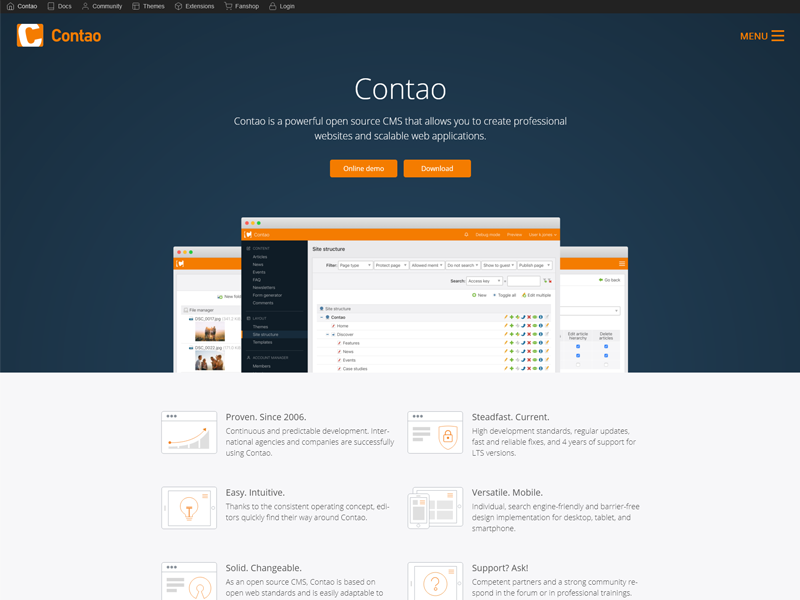This is a screenshot from the website Kontau. The header prominently displays the name "Kontau" twice: once at the top left corner featuring the brand's icon—a bolded "C" in an orange square—against a very dark blue, almost dark gray, background, and again at the top center in large white letters followed by a tagline in smaller white text. The tagline reads, "Kontau is a powerful open-source CMS that allows you to create professional websites and scalable web applications." Below this description, there are two orange buttons labeled "Online Demo" and "Download."

The image showcases three browser windows displaying different aspects of Kontau, including its site structure and other features for scalable website management. Below this main section, the page transitions to a light gray background divided into six sections, each highlighting different attributes of the app. These sections are accompanied by charts or icons and are titled: “Proven since 2006,” “Easy & Intuitive,” “Solid & Changeable,” “Steadfast & Current,” “Versatile & Mobile,” and “Support & Ask.”

Additionally, the website's menu is situated at the top right corner, indicated by three horizontal lines in orange.